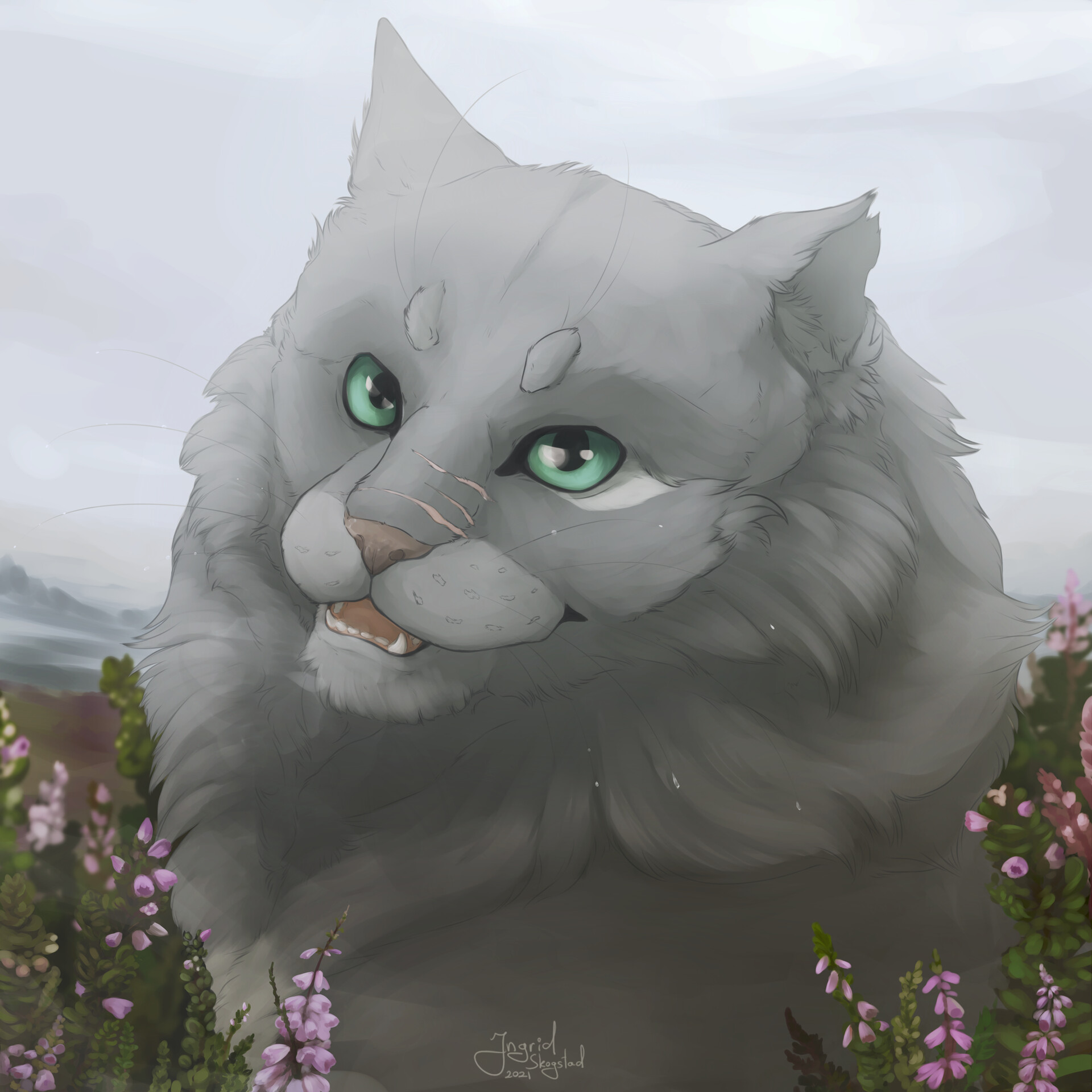This slightly rectangular image showcases a detailed drawing, possibly a painting, of a long-haired gray cat with a thick mane. The cat, which has light green eyes and a pink nose, is depicted facing toward the left but with its head slightly tilted to give a more frontal view. Its fur is a mix of gray shades, with the fur around its mouth being a lighter gray. The cat is standing in a field filled with green plants and pink wildflowers that surround it, complemented by a cloudy gray sky and distant gray mountains in the background. Small snowflakes are softly floating around its neck. At the bottom center of the image, there is a small, somewhat hard-to-read signature in white cursive text, which reads "Ingrid Skogstad, 2021." The cat’s mouth is slightly open, revealing its teeth, including one visible canine tooth. Additionally, there are three small scratches on its nose.